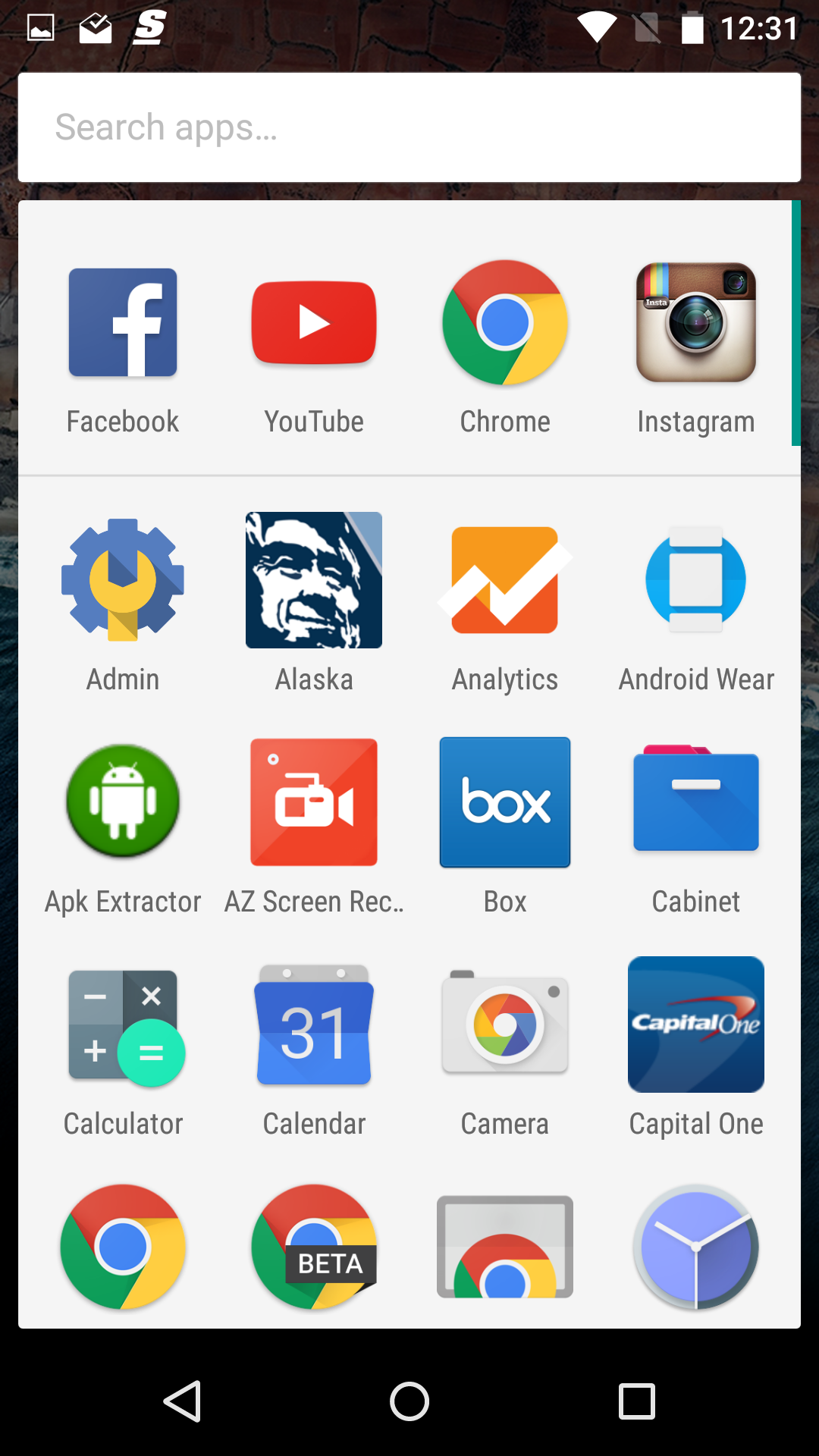The image depicts a black rectangular screen, most likely a smartphone home screen. 

In the upper left corner, there are white-outlined signal bars and small hill icons, indicating cellular network strength. Adjacent is a square icon with a checkmark on top, likely a notification or status indicator. Not far from there is an "S" with an underline, potentially a shortcut or special key.

On the right side of the screen, there's a Wi-Fi icon indicating the connection status, next to which is a light gray rectangle with a crossed-out battery symbol, possibly indicating battery status. Below this, the time is displayed as "12:31". 

Dominating the rest of the screen, there are two white rectangular search bars. The top one says "Search apps" and below that is another white rectangle, prevalently indicating a list of apps on the device. 

The visible apps, from left to right and top to bottom, include:

- Facebook: Recognizable by its blue icon with a white "f".
- YouTube: A red rectangle with a white arrow pointing right.
- Chrome: Displaying the iconic colorful circle.
- Instagram: Depicted by a camera icon.
- Admin: Represented by a gear symbol.
- Alaska: A blue face avatar.
- Analytics: An icon resembling a graph.
- Android Wear: A white circle with a blue piece of film.
- APK Extractor: A green circle with a robot icon.
- AZ Screen REC: An orange square with a video camera.
- Box: A blue box with the word "box" in white.
- Cabinet: A blue drawer with a white handle and pink tabs peeking out.
- Calculator: A classic calculator icon.
- Calendar: A blue page of a calendar.
- Camera: Standard camera icon.
- Capital One: A blue square with the red Capital One swoosh.

Further, there is an icon of Chrome repeated twice, one of which is branded with a gray rectangle that says "beta". Next to this is another icon that looks like a screen displaying part of the Chrome symbol.

Lastly, there's an interesting icon outlined in gray and filled with dark purple on the left and lighter purple on the right, featuring three lines. Below it are media control icons: a left-pointing triangle, a circle, and a square, suggesting playback control functions.

This detailed view provides a comprehensive look at the smartphone's main display, reflecting a typical, organized arrangement of frequently used applications and status indicators.